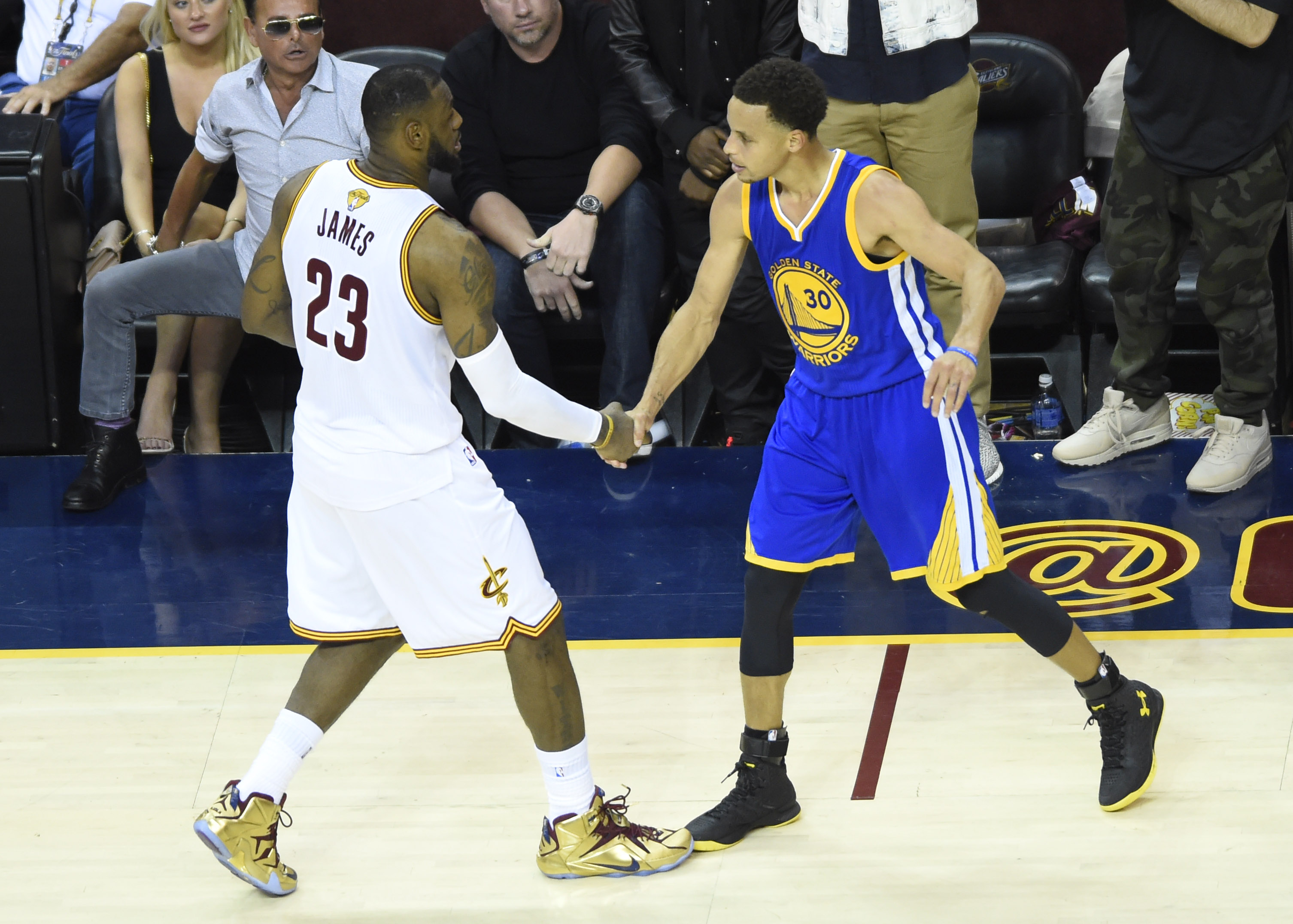In a professionally taken photograph, two African-American basketball players are captured shaking hands on an indoor court, likely in the middle of a game. The player on the left, possibly LeBron James, wears a white uniform adorned with maroon and gold details, with 'James' and the number 23 on the back. He has darker skin, a goatee, tattoos on his arms and legs, and is sporting golden sneakers. The opposing player stands on the right, dressed in a bright blue jersey with yellow and white accents, showcasing the number 30. This player, who has lighter skin and no visible tattoos, wears black sneakers. Behind them, a few rows of the crowd are visible, including a man with sunglasses and a light shirt, a blonde woman, and another man in a black shirt. The court itself features maroon, gold, blue, and white markings, and an ax symbol is slightly visible. The image overall highlights a moment of sportsmanship as the players face each other in a handshake.